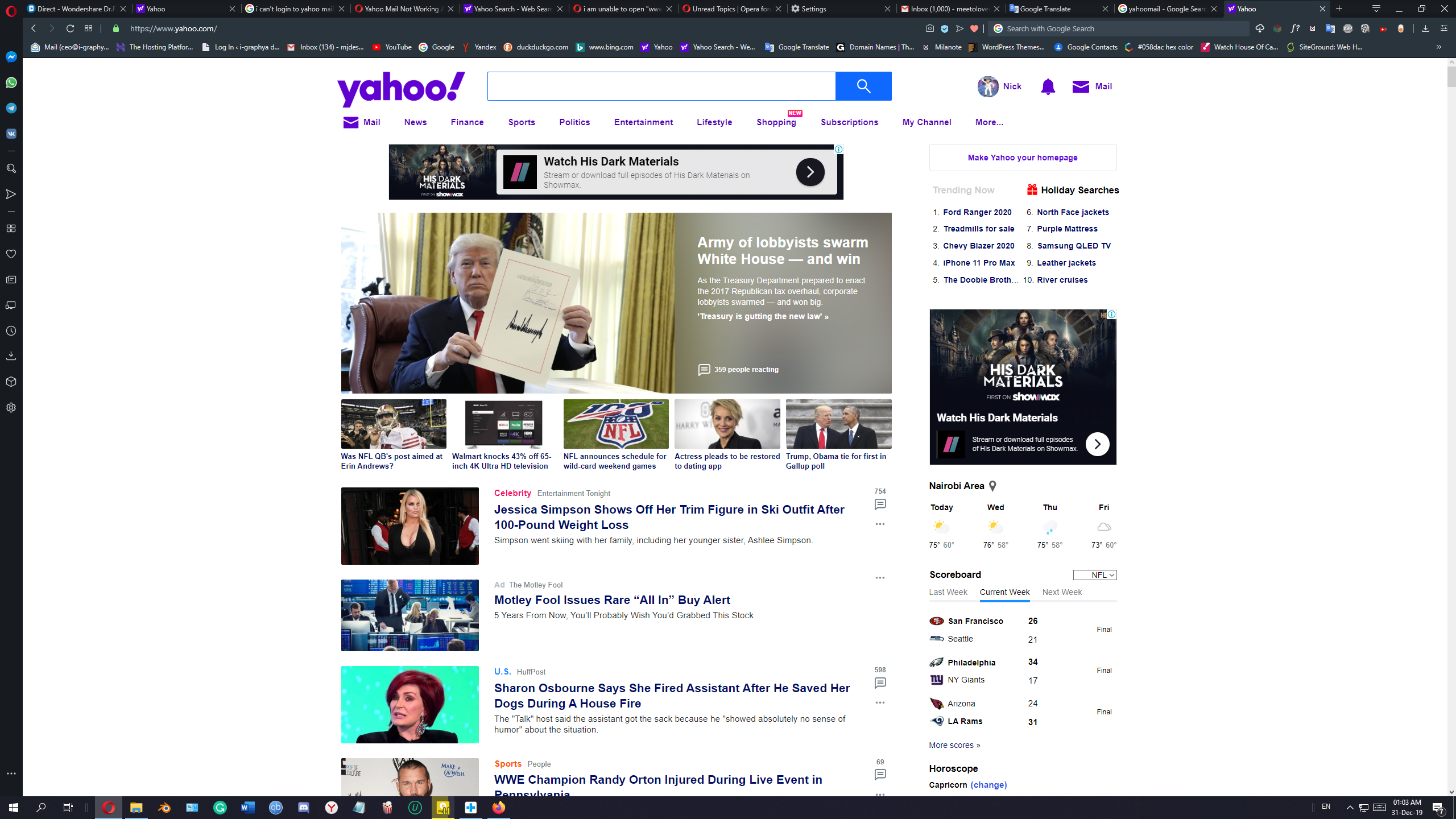**Detailed Caption:**

This is an image of a computer screen displaying a web browser with multiple tabs open, stretching across the entire top bar. The URL in the search bar is "https://www.yahoo.com," indicating that the Yahoo homepage is being displayed. Directly below the search bar, there are additional browser bookmarks, though they are too small to decipher clearly.

On the left side of the webpage, there is a narrow navigation bar filled with various icons. From top to bottom, these icons include a blue one, a green one, two more blue ones followed by a divider line, a magnifying glass, a play button, a grid of squares, a heart, a pair of overlapping squares, and several other indistinguishable icons.

The main content area shows the Yahoo homepage, prominently featuring the Yahoo logo in purple at the top. Below the logo, there is a search bar and a series of navigation tabs labeled: Mail, News, Finance, Sports, Politics, Entertainment, Lifestyle, Shopping, Subscriptions, My Channel, and More.

At the top right of the page, there is a profile section with a small image that reads "Nick," alongside an icon of a Lorne Bale, which represents the user. An advertisement for a TV show is visible beneath this profile section.

The central portion of the page displays a list of news articles. The first article features an image of Donald Trump seated and holding a paper, with the headline "Army of Lobbyists Form White House and Win." Below this is another news section related to the NFL, showcasing a 49ers player and an NFL logo on the field. 

Following that, there are images of a blonde actress standing next to Trump and Obama, as well as an article headline about Jessica Simpson: "Jessica Simpson Shows Off Her Trim Figure in Ski Outfit After 100-Pound Weight Loss." Another article mentions that "Motley Fool Issues Rare All-In Buy Alert," accompanied by an adjacent image.

The final visible article headline reads, "Sharon Osbourne Says She Fired Assistant After He Saved Her Dogs During a House Fire," showing an image of Sharon Osbourne against a green backdrop.

To the right of these articles, there is an advertisement for a show titled "Historic Materials," alongside some trending topics that are unreadable due to the small text. Further down, a weather section and an NFL scoreboard are displayed. The background of the entire site is white, providing a neutral backdrop for the diverse content.